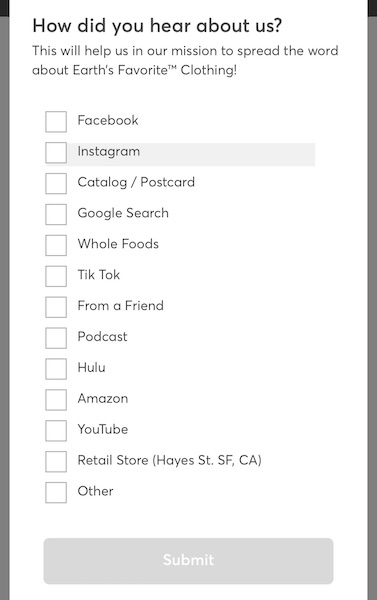This image is a screenshot captured in portrait mode. It showcases an online form meant for gathering customer feedback. The background consists of diagonal gray stripes extending from the upper left to the lower left and from the upper right to the lower right. 

In the upper left corner, there is a black rectangle, mirrored by another black rectangle in the upper right corner. Overlaying the upper right black rectangle is a white text box with the prompt in black font: "How did you hear about us?" followed by a supplementary message in gray font: "This will help us in our mission to spread the word about Earth's favorite clothing!"

Below this text are multiple categories, each accompanied by an unchecked checkbox. The categories listed are: Facebook, Instagram, catalog, postcard, Google search, Whole Foods, TikTok, From a Friend, podcast, Hulu, Amazon, YouTube, retail store (Hay Street, San Francisco, California), and other. Notably, the Instagram option has a gray background, suggesting the cursor is currently hovering over it and is about to select it.

At the bottom of the form, spanning from the bottom right to the bottom left, is a large gray button inscribed with "Submit" in small, white font. The size of the button contrasts with the small text, making the call-to-action somewhat difficult to read against the gray background.